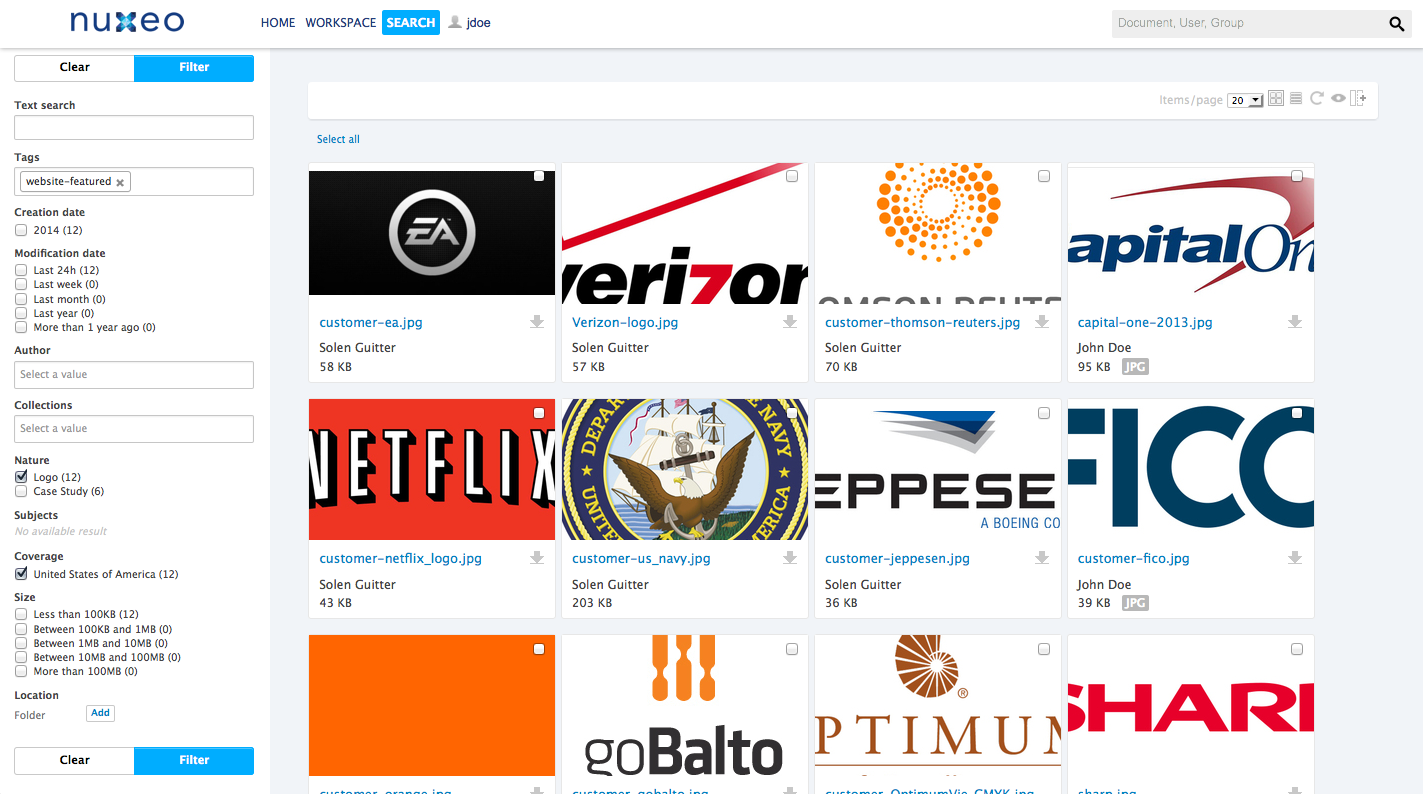This image captures a detailed view of a web interface for a platform branded as "Nuxio." Dominating the top of the interface is a white border separated by a thin, grayish-black horizontal line. Within this border is the "Nuxio" logo, featuring "Nuxio" spelled out in blue with a distinctive "X" that has a gradient from dark blue to light blue at its center. Adjacent to the logo are navigation options in blue font, labeled "Home" and "Workspace," along with a blue search rectangle housing white text and a user icon labeled "J. Doe."

In the top right corner, users can find a search bar represented by a magnifying glass icon. On the left side of the interface, a vertical toolbar provides functionalities such as "Clear" and "Filter," with the word "Filter" prominently displayed in blue with white lettering. This toolbar includes various search options and settings for modifications.

Central to the webpage is a large gray area containing a search bar at the top. Below the search bar, a grid-like structure lists several apps and programs, including "Customer EA," "Verizon," "Capital One," "Netflix," "Scion Center," and "Sharp," among others. This section appears to offer users the ability to search for and navigate through different applications or icons. At the top of this section, additional options are available for filtering and toggling the view between grid and list formats, as well as other modification settings.